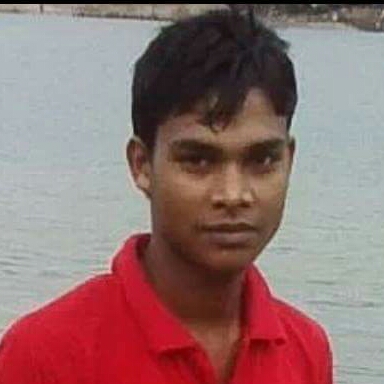This color photograph, possibly from the 1980s or 1990s, features a young man of Indian or Southeast Asian descent with dark skin and black hair styled swooped to the left on his forehead. He is wearing a perfectly pressed red polo and is visible from his head to just below his shoulders. The image has a slightly grainy texture, adding to its aged appearance. The young man has a piercing, almost expressionless, and somewhat annoyed stare directed at the camera. His nose is flared slightly, and his rounded ears are noticeable. He stands against a backdrop of a light aqua-colored body of water, possibly a lake or a bay, with the faint outline of land structures along the top edge of the image, suggesting a distant city line. The water appears to be in motion, hinting at a colder day. This photograph embodies a style of photographic realism and representationalism.